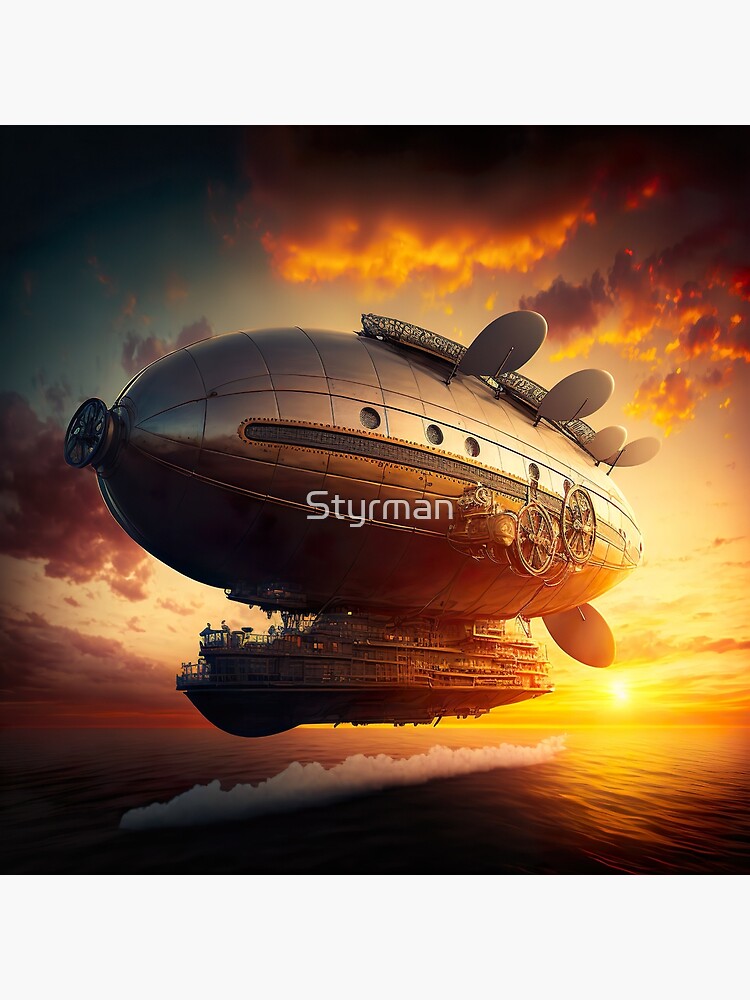The image depicts a digital illustration of a futuristic, chrome-plated sky blimp divided into cube-like sections. The large, tan balloon part of the blimp features white lettering spelling out "S-T-Y-R-M-A-N." Fitted with what appear to be sails or solar panels, the blimp has a wheel mechanism at the front, likely used for propulsion or steering. Attached below the blimp is a multi-storied structure resembling a cruise ship, approximately three or four stories tall.

The scene is set outdoors during either sunrise or sunset, casting a striking orange glow throughout the image. The blimp, positioned centrally and angled left to right, hovers over an ocean devoid of land masses. The ocean surface shows white streams and splashes, possibly indicating recent takeoff or imminent landing. The sky above is a mix of moderate clouds in hues of yellow, orange, black, gray, and light blue, with the clouds catching the sunlight and creating a spectrum of warm tones. The setting emphasizes the fantastical nature and detailed craftsmanship of the illustration.